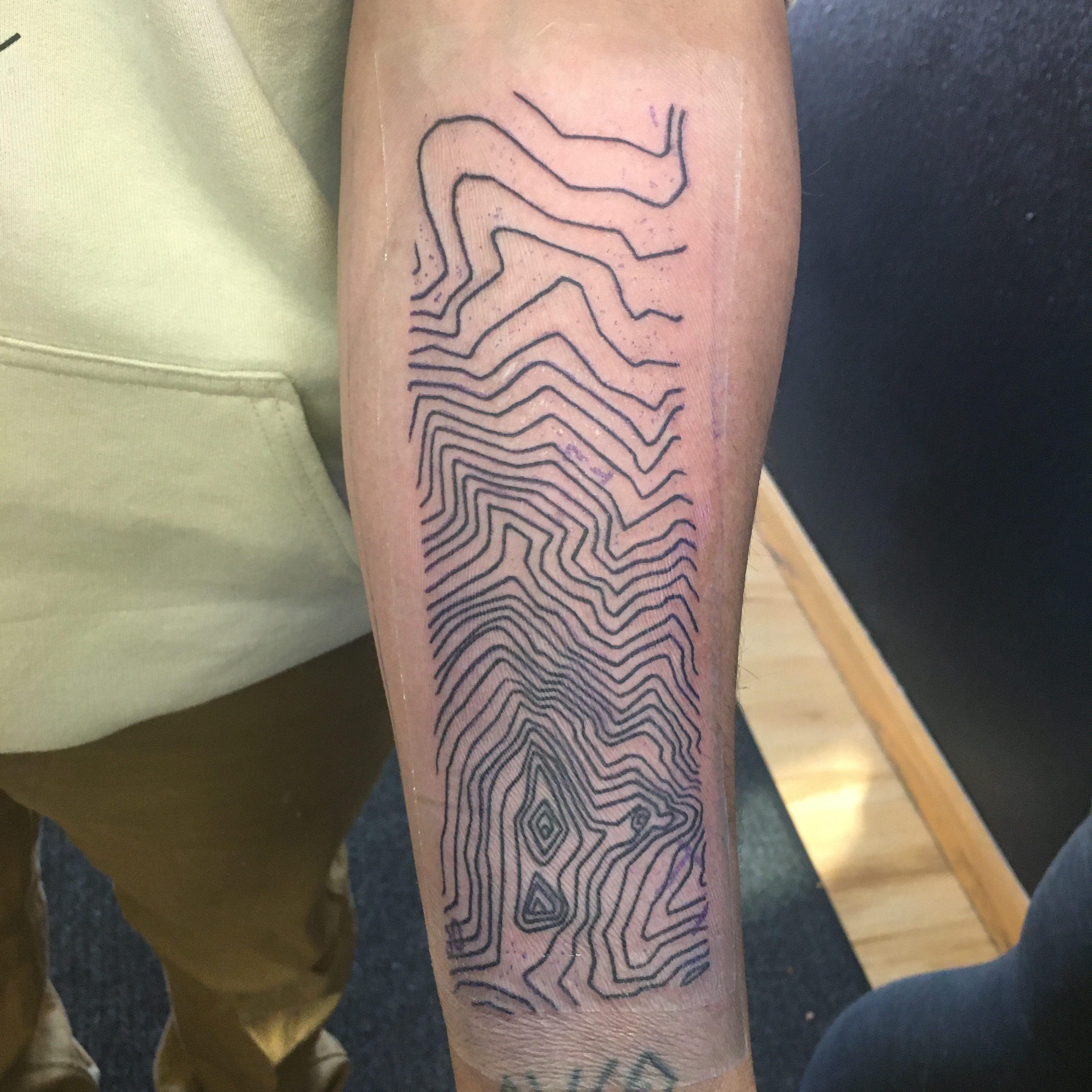The photograph captures a close-up of a person's left forearm, prominently showcased in the center of the image. The arm is stretched vertically, revealing a freshly inked tattoo that spans from just above the wrist to just below the elbow. The wearer is dressed in a light yellow hoodie, visible around the hand pockets and the lower half of the garment. The tattoo itself is an abstract design, reminiscent of a topographical relief map or a wood grain pattern with intricate, squiggly lines and expanding rings emanating from a central point. The tattoo, etched in black ink, covers most of the inner forearm and shows signs of freshness, including a protective paper and surrounding redness. In the background, there's a blue wall and a floor with blonde oak flooring adjacent to carpeting. The scene is carefully framed to highlight the detailed and unique characteristics of the new tattoo.